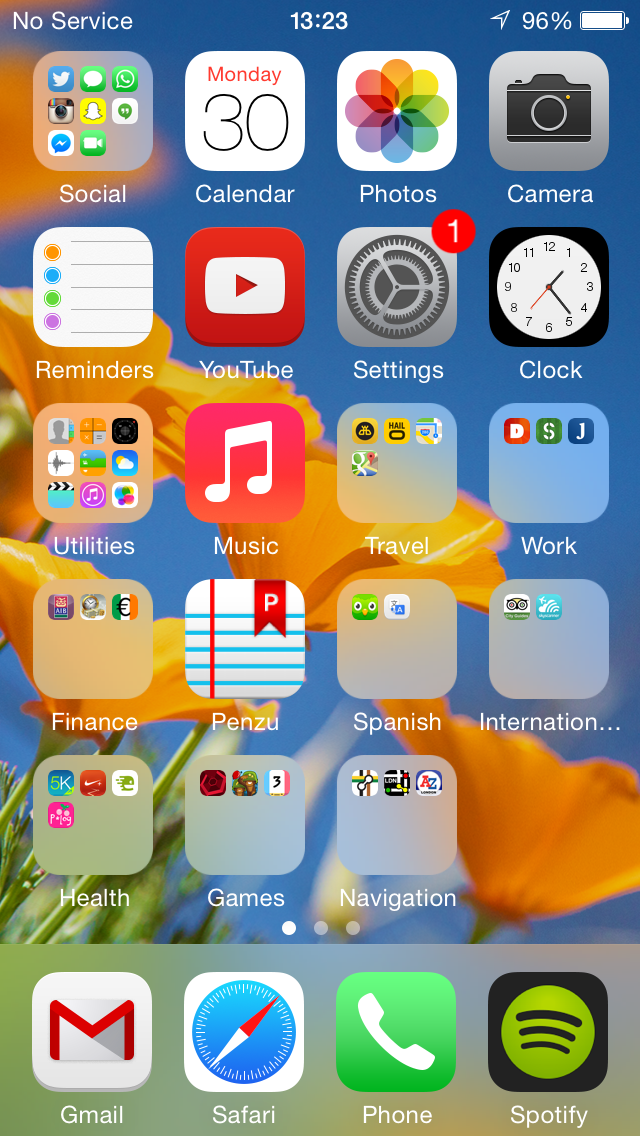This image is a screenshot of a cell phone's home screen. The screen's aspect ratio is taller than it is wide. The background is an outdoor shot taken during the daytime, prominently featuring vivid orange flowers that stretch diagonally from the lower left corner towards the upper right edge of the screen. 

At the very top, in small text, the notification bar reads "No Service". Below this, centered on the screen, is the time displayed as "13:23". To the right of the time, an icon shows a battery at 96% charge, with an arrow beside it.

The home screen is organized into four columns and four rows of app icons, totaling 16 apps, with an additional three apps on the bottom taskbar, making a total of 19 apps visible. The taskbar features the icons for Gmail, Safari, Phone, and Spotify.

The apps appear standard and not customized, except for the "Social" folder containing various social media applications. The visible apps include Calendar, Photos, Camera, and other default phone apps. There are also folders labeled "Utilities," "Travel," "Work," "Finance," and "Spanish," the latter of which contains Duolingo and another language-learning app. Other notable apps include a Penzu notebook app, an international health app, games, and navigation tools.